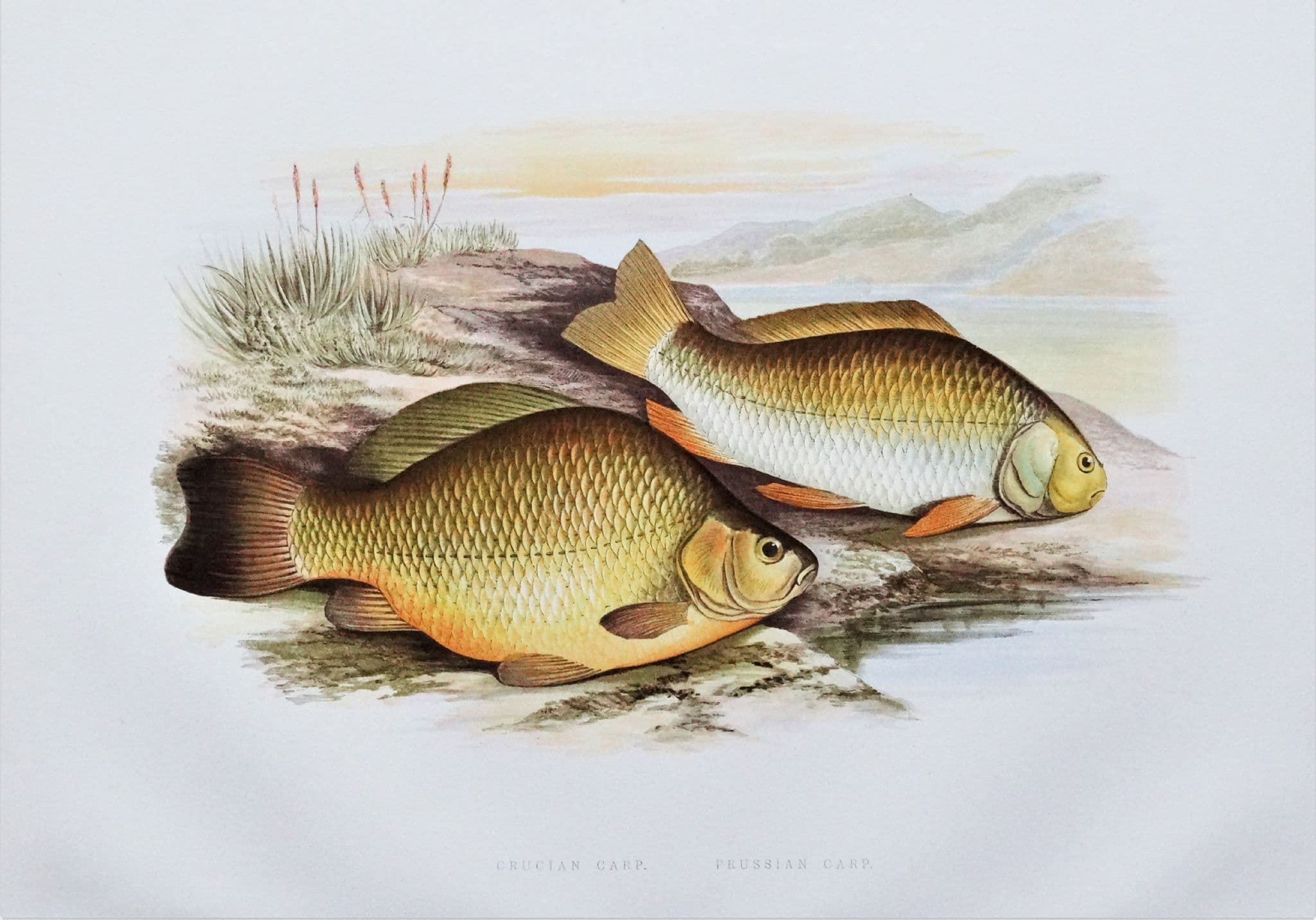This artwork is an intricate drawing and painting depicting two fish on land, situated near a lake with an expansive, light blue sky above, accented by clouds tinged with an orange hue from the setting sun. The fish are positioned on a rock or bank covered with sparse plant life, including grass and weeds, against a backdrop of serene hills or mountain ranges. The scene is rich with hues of orange, green, blue, and brown—the fish boast gold and white scales with gold and brown fins. The larger fish occupies the bottom left or middle left section of the painting, while the smaller, narrow fish is found in the top middle section. Both fish are oriented towards the water, as if longing to return. The scene is enclosed within a vignette, leaving a prominent white border around the artwork. There is also an indistinguishable signature or marks at the bottom, adding a personal touch to this compelling piece.